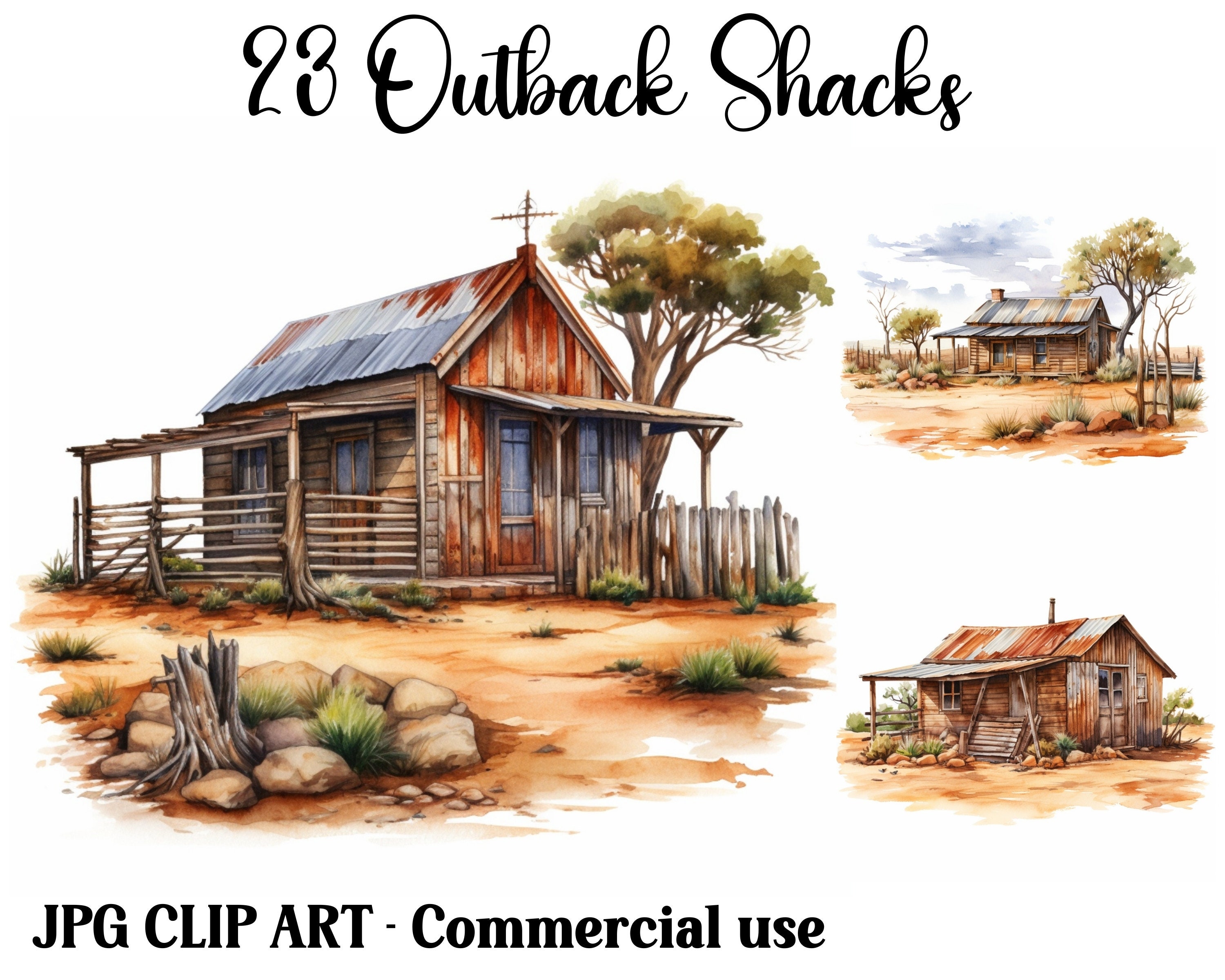This image depicts a piece of clipart labeled "23 Outback Shacks." It features three animated shacks on a white background, each illustrating different perspectives of what could be the same wooden outback shack. The primary shack on the left is a small wooden structure with a large cross on its roof, a fenced-in yard, and a tree beside it. In the foreground, there are rocks and patches of grass scattered around, enhancing the deserted outback ambiance. The additional two shacks on the right are similar, potentially showcasing different angles or variations. The second shack is surrounded by multiple trees, while the third is flanked by bushes. At the bottom, the label "JPG Clipart-Commercial Use" indicates that this image is intended for commercial purposes.